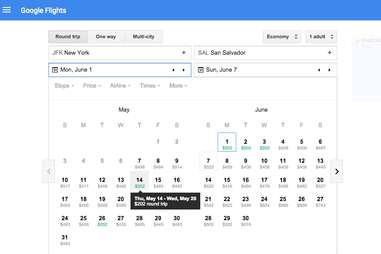The image is a screenshot of a Google Flights page with a distinct blue border across the top. On the top left, there are three horizontal white lines stacked atop each other, and the words "Google Flights" are displayed in white against the blue border. Below this header are two side-by-side calendar views for the months of May and June.

The image quality is blurry and out of focus, making some text difficult to read. At the top of the calendars are tabs labeled "Round-trip," "One-way," and a third tab that is partially illegible, possibly saying "Multi-city." Directly below the tabs, the departure airport is listed as "JFK New York" and the arrival airport as "SAL San Salvador."

Beneath these details, on the left side, there is a calendar icon with "Monday, June 1" next to it, and another calendar icon on the right with "Sunday, June 7." The left calendar corresponds to May and shows the days of the week at the top, abbreviated to single letters (e.g., M for Monday). May starts on a Friday (the 1st), with dates 1 through 6 printed in a lighter typeface, while the 7th through the 31st are in darker, bold type. The 14th of May is highlighted and subtitled with the out-of-focus text "Thursday, May 14 to Wednesday, May 27." Below this subtitle, the text is too blurred to decipher.

The right calendar displays the month of June. It similarly starts with days of the week labeled across the top, showing that the 1st of June falls on a Monday. The only date marked in June is the 1st, which is outlined with a square.